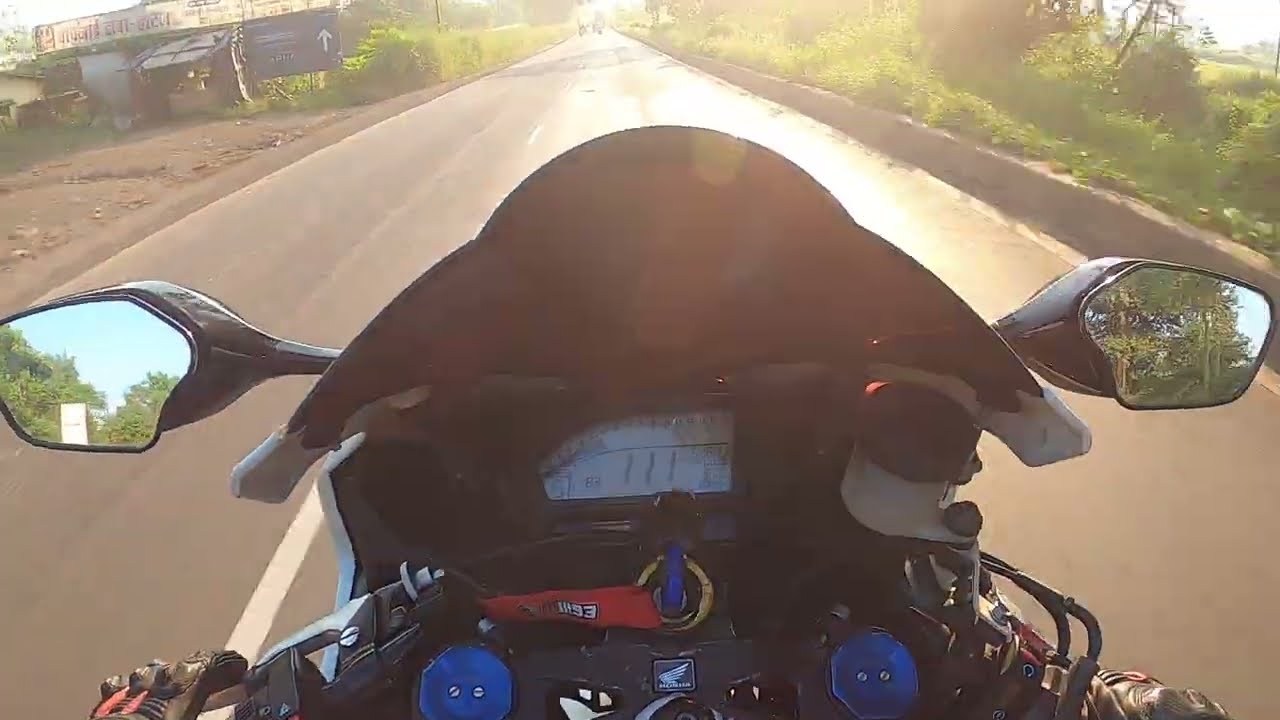The image captures a vibrant and immersive point of view from a motorcyclist. Dominating the center, the motorcycle's dash is in clear focus, showcasing a sleek and detailed layout. Both of the motorcyclist's hands, clad in dark brown, black, and orange gloves, grip the handlebars firmly. The dead center of the dash features a distinctive blue key with a long red keychain attached, flanked by blue circular indicators on either side. Just above, a computerized speedometer reads 111, possibly indicating speed. The surrounding environment is brightly lit by intense sunlight, necessitating a squint to look ahead. On either side of the motorcyclist stretches a single-lane road framed by rural scenery, including trees, bushes, and a mix of run-down buildings to the left. Reflections of the serene blue sky and trees can be seen in the rearview mirrors, enhancing the sense of motion and journey in this sunny, midday ride.